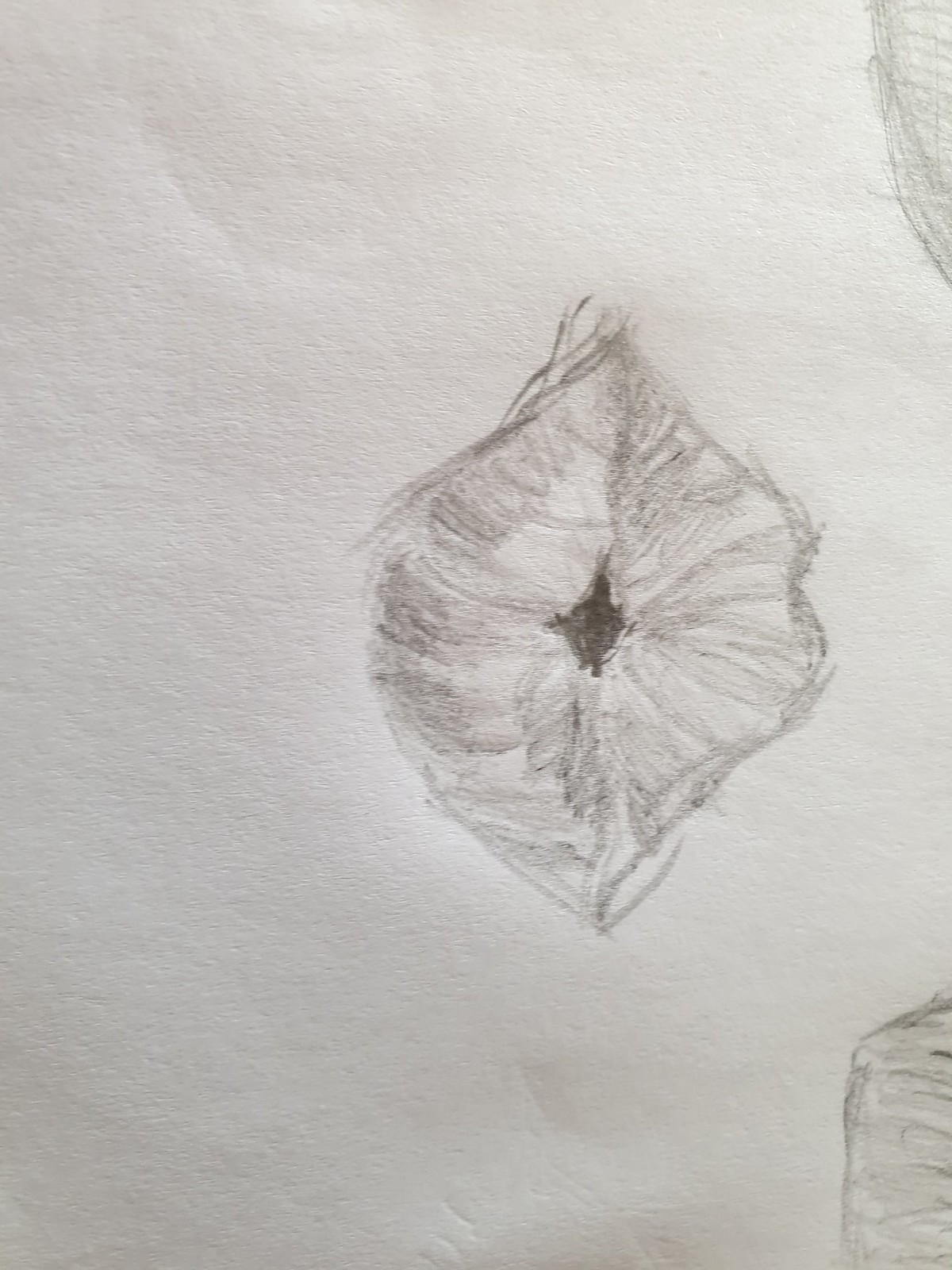This detailed black and white drawing, created with charcoal pencil on a white piece of paper, prominently features a pair of lips oriented sideways and centrally positioned. The lips are scrunched together, resembling a kissing gesture, with a distinct black shading in their center adding depth and contrast. On the right-hand side of the paper, there are two additional sketches. The lower sketch is more discernible, appearing to be a square, while the upper sketch remains ambiguous and harder to identify.